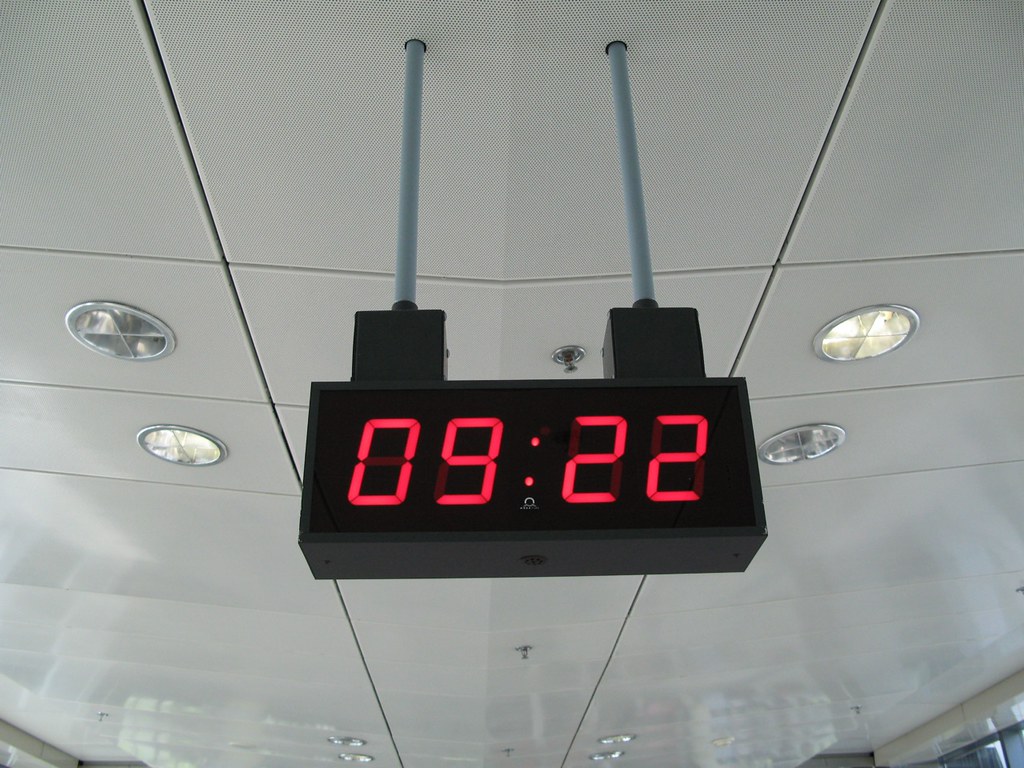In this horizontally oriented rectangular photograph, the viewer's perspective is directed towards a white, typical drop ceiling, known for its grid-like pattern of tiles. The ceiling features several light fixtures, softly illuminating the scene. The focal point of the image is a black-backed digital clock mounted in the center. This clock is suspended from the ceiling by two silver poles, attached via small square brackets. The clock prominently displays the time "09:22" in bright red digital digits. Additionally, in the lower right corner of the photograph, there is a partial view of the top of a window pane or a glass door, which hints at a larger architectural space beyond the immediate ceiling view.